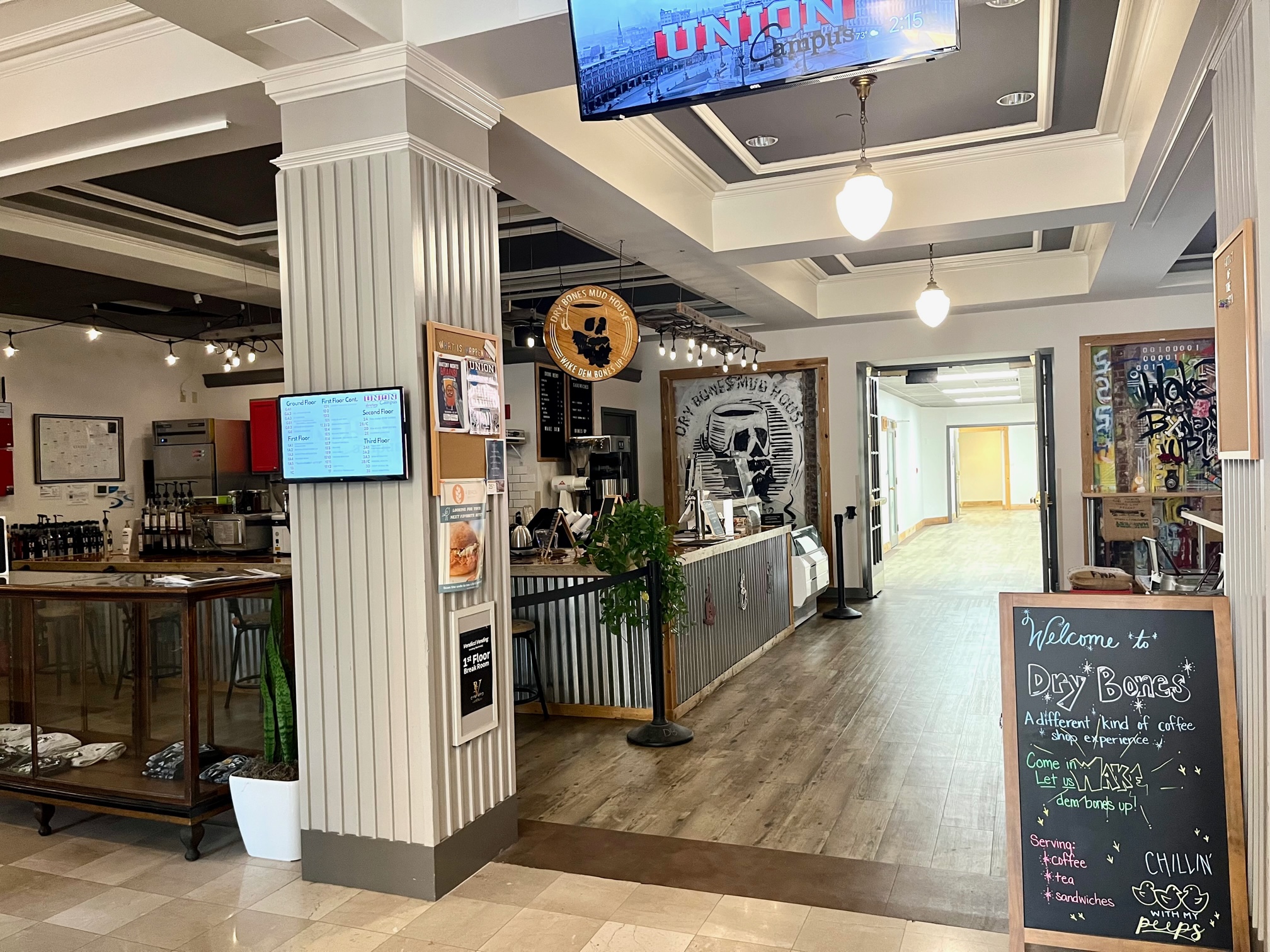This detailed and vivid photograph captures the inviting interior of "Dry Bones," a distinctive coffee shop likely situated within a larger building, such as a university campus or a library. The image is a horizontal rectangle, showcasing a charming and cozy atmosphere that blends rustic and modern elements.

In the bottom right-hand corner of the photo stands a prominent chalkboard sign framed in light brown wood, welcoming patrons with playful chalk writing in various colors. It reads: "Welcome to Dry Bones, a different kind of coffee shop experience. Come in, let us wake dem bones up. Serving coffee, tea, sandwiches, chillin' with my peeps," accompanied by cheerful chalk drawings of little chickens.

On the left side of the image is the main coffee bar countertop, clad in wood with a rustic tin sheeting, creating a warm contrast against the sleek coffee-making equipment in the background. Various syrup bottles with pumps and modern appliances line the countertop, hinting at the array of beverages available. A TV monitor mounted above displays the words "Union Campus," suggesting the shop's connection to a university.

A central pillar in the shop adds to the decor with bulletin boards and signage pinned on it. Nearby, a wooden display case showcases neatly folded t-shirts, contributing to the shop's unique merchandise offerings. The floor transitions from a tan wood near the front to cream-colored tiles in the background.

Hanging above the bar area is a round sign, and an eye-catching black and white wall sign at the rear announces "Dry Bones Mug House" with a stylized skull image, reinforcing the café’s playful branding. The ceiling features a mix of black and white colors, with pendant lights adding a touch of modern charm.

The far end of the shop features a bright hallway leading to other parts of the building, suggesting a spacious and well-connected environment. An array of posters and announcements decorate the walls, ensuring the space feels lively and community-focused.

Overall, Dry Bones appears to be a well-designed, inviting place for students and visitors to relax, enjoy refreshments, and engage with a vibrant campus community.